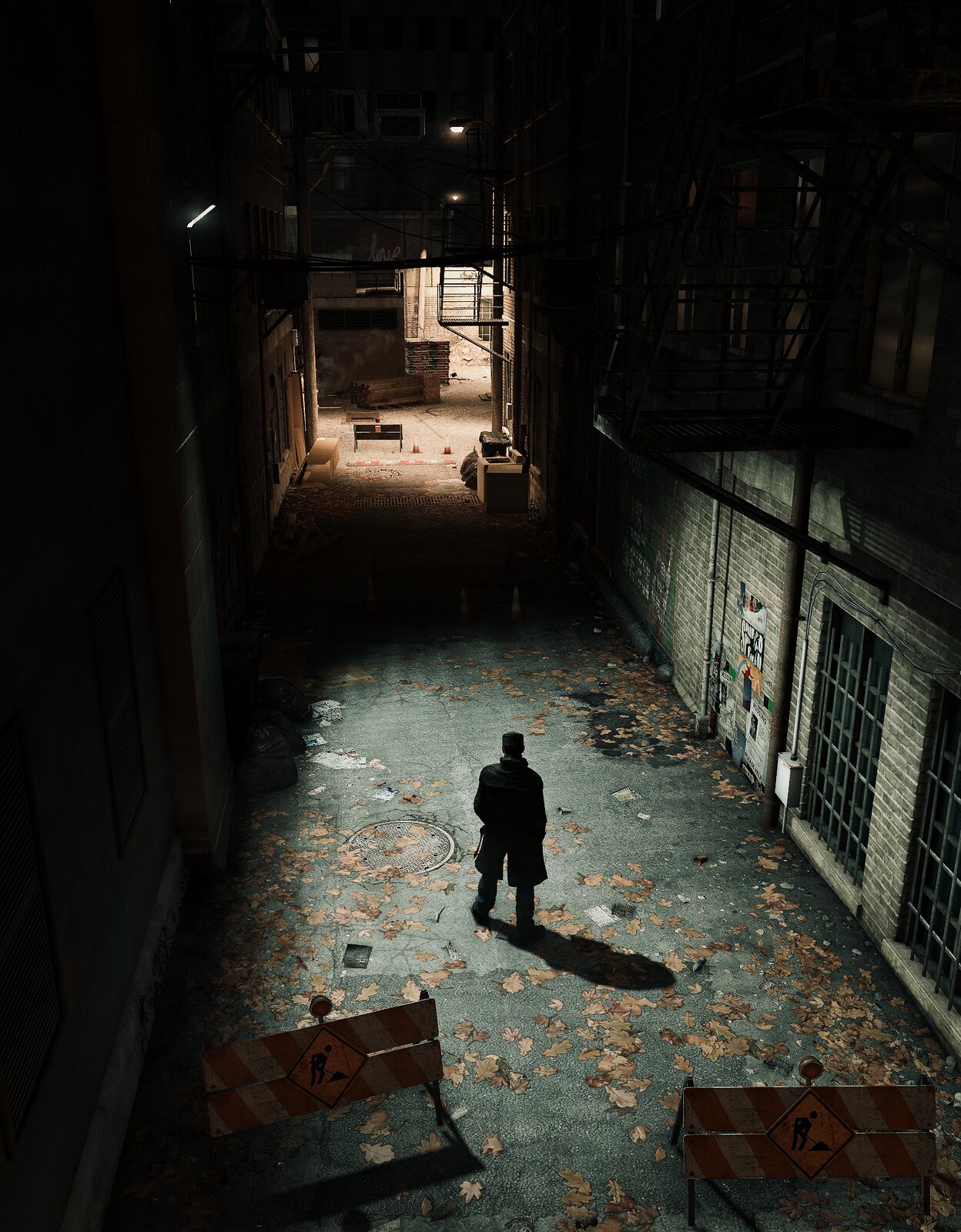The image is a vertically aligned, aerial view of a slightly downward-slanting alleyway that has fallen into disrepair. The ground is littered with a mixture of trash and stepped-on light orange leaves. Positioned close to where the image was captured are two orange and white striped construction signs featuring an image of someone digging or shoveling, effectively blocking off the alley. Dominating the right side of the alley is a gray brick wall with what appear to be iron doors, though they likely do not open. In the center of the alleyway stands a man dressed in a long, black coat, visible from behind and casting a shadow, while being illuminated by a nearby light. The alley stretches towards an industrial-looking space with a large open doorway, where light from the street beyond filters in with a brownish hue, adding to the scene's eerie and neglected atmosphere.